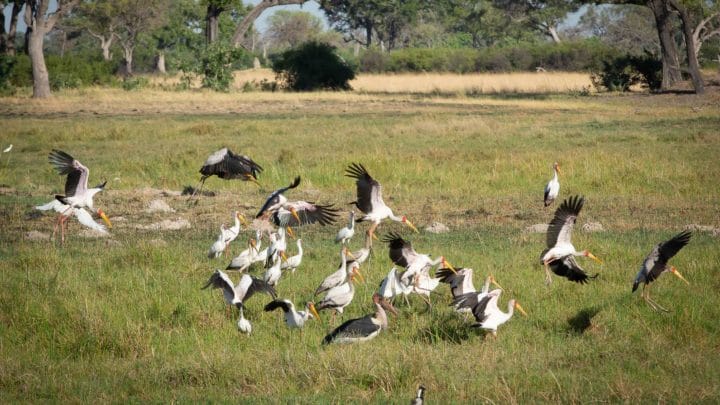In this image, you see a lively scene of a flock of about 20 to 25 large birds with striking white bodies and black and gray wings, accented with long, yellow beaks. The birds are both flying and walking around an expansive grassy area, which features patches of green, yellowish, and somewhat burnt looking grass. Some birds are seen with their wings folded, standing tall on long legs, while others are either flapping their wings just above the ground or are in full flight. The background is adorned with a variety of trees, bushes, and hedges, providing a lush, natural setting under a clear blue sky. The scene captures the dynamic motion of the birds as they appear to be moving towards an unseen destination, creating a sense of lively activity amid the grounded and aerial fluttering of their wings.